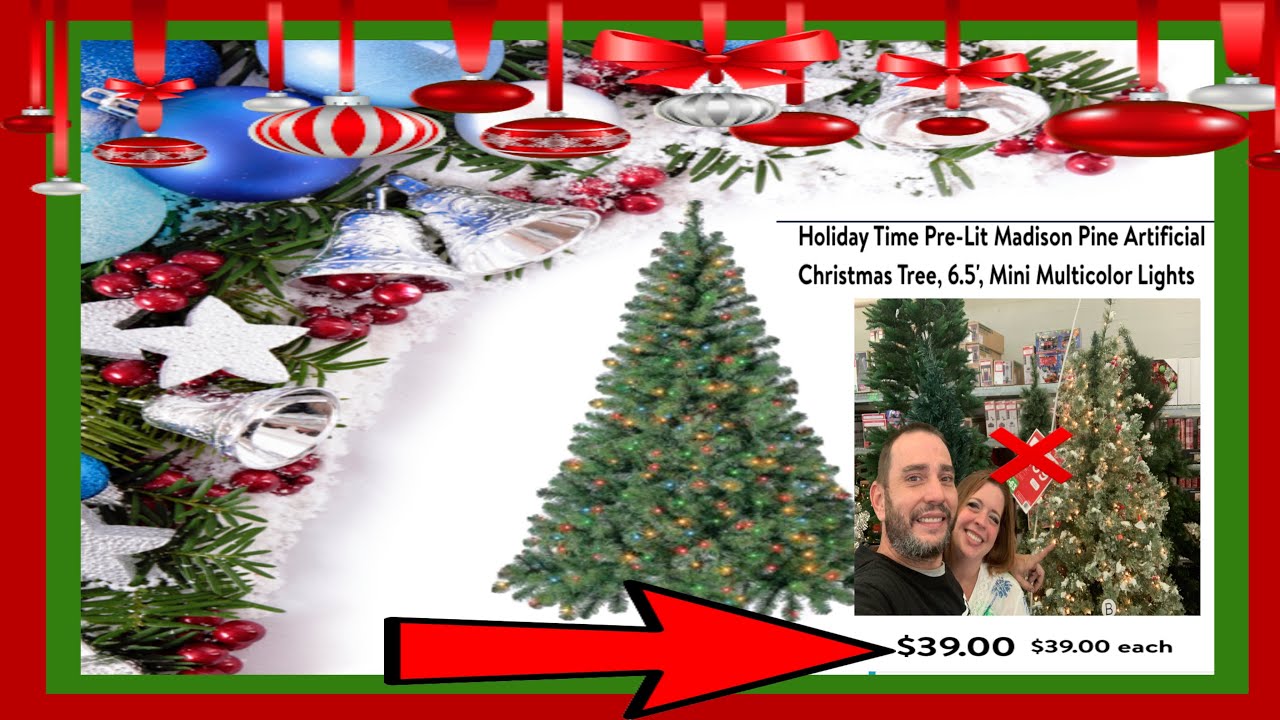In this rectangular image, a cheerful man and woman are located on the right side, both smiling warmly. The woman, with her brown hair, is dressed in a white and blue top. Next to her stands the man, who has a distinctive black and white beard and mustache, and is wearing a black outer shirt over a gray inner shirt. Behind them, several Christmas trees create a festive backdrop. Prominently featured in the center of the image is a decorated green Christmas tree adorned with multi-color lights, adding a vibrant touch to the scene. At the top of the image, text reads, "Holiday Time Pre-Lit Madison Pine Artificial Christmas Tree, 6.5 feet, many multi-color lights." Below, a large red arrow from the left points to the text "$29 each," indicating a price promotion for the trees.